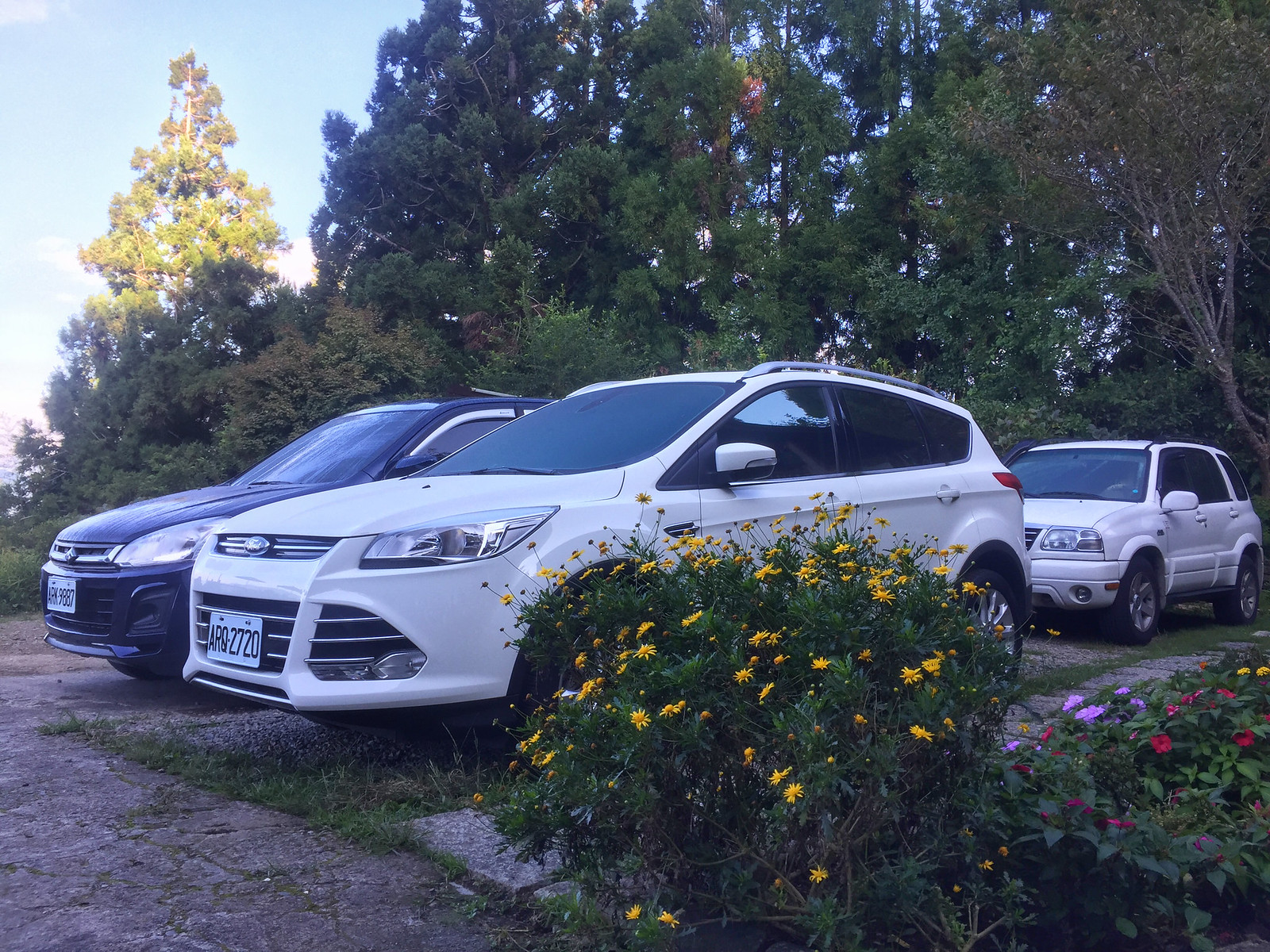This image captures a parking area adorned with natural foliage under a partly blue sky with wispy clouds. In the foreground is a white, four-door car with an oval logo on the front grille, and a front license plate, parked facing left. Parallel to this car is another vehicle, similar in size and shape, painted dark blue or black. Both cars are parked on what appears to be cracked cement with patches of gravel and grass, suggesting an improvised parking lot. Behind the front white car, partially obscured, is another small white four-door CUV, facing the same direction.

Surrounding the cars, the scene is lush with greenery. To the front right side of the image, a vibrant green bush blooms with an abundance of small yellow flowers. Further to the right of this bush, there's a mix of smaller green plants dotted with pink, purple, red, and a few yellow flowers. The backdrop is a lush array of trees; a mix of evergreen and deciduous, exhibiting varying shades of green. This natural setting creates a serene and picturesque background to the parked vehicles.